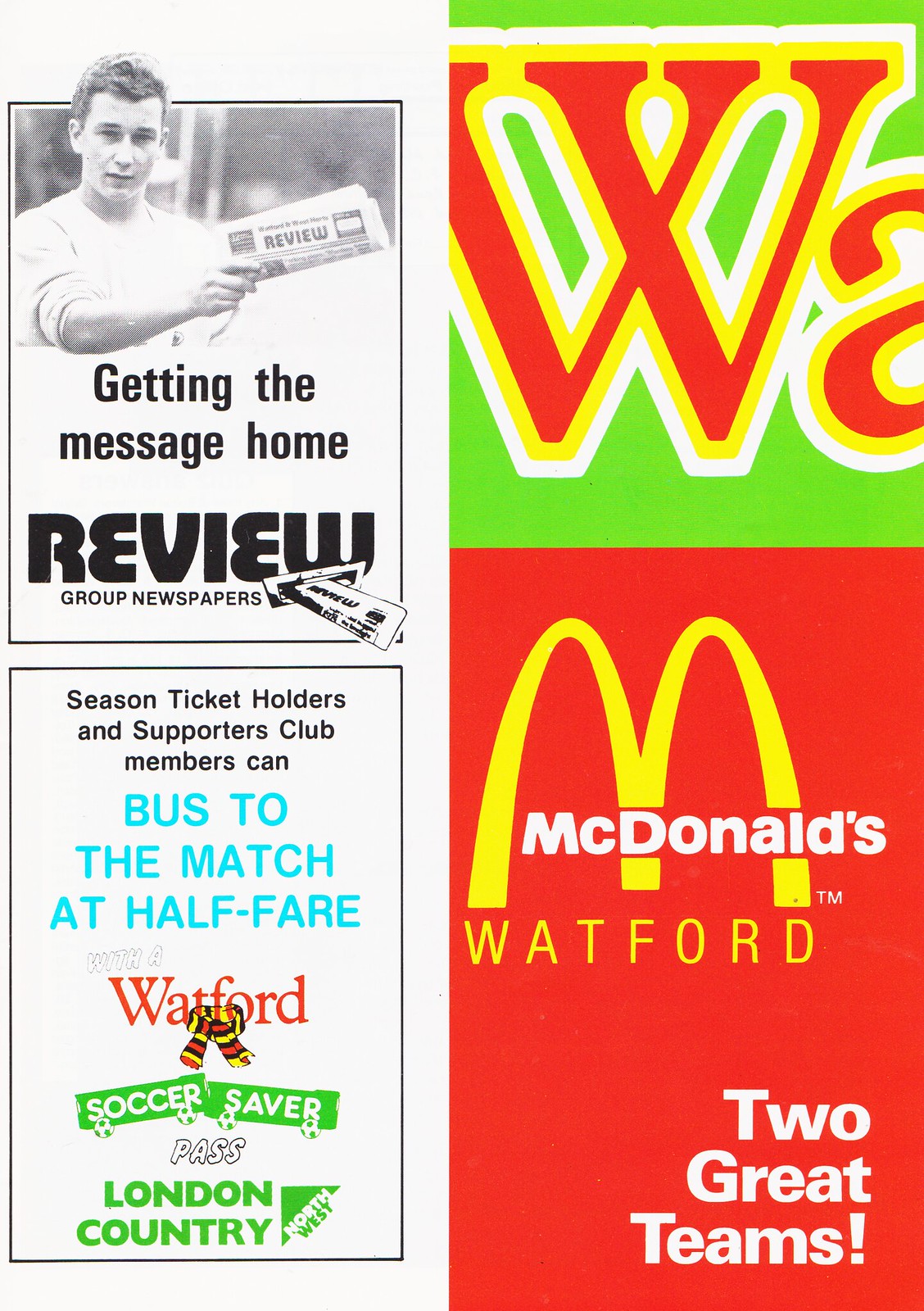The image is a scan or photograph of a page containing four advertisements arranged in a grid with two ads on the top row and two on the bottom row. 

In the top left corner is a vertical, black-and-white ad showing a young Caucasian man with light brown hair holding a folded newspaper in his right hand while wearing a white T-shirt. The text below his extended arm reads "Getting the Message Home" in black letters, followed by "Review" in bold black text, and "Group Newspapers" in smaller black text. There is a small graphic of a newspaper entering a mail slot below the text.

Directly below this, in the bottom left corner, is an ad aimed at sports fans. It starts with black text reading "Season Ticket Holders and Supporters Club Members Can," followed by blue text stating "Bus to the Match at Half Fare." Beneath this, "Watford" appears in red text next to a soccer logo, followed by a green banner with "Soccer Saver," and then the word "PASS" in bold outlined text. The bottom part of the ad features "London Country" in green sans-serif lettering beside a green and white square logo.

On the upper right corner is a square ad with a green background showcasing large red letters "W" and "S" (the "S" is cut off) outlined first in yellow and then in white.

In the bottom right corner, a McDonald's ad with a red background displays the familiar McDonald's golden arches logo at the top left, with the word "Watford" underneath in yellow text. The ad concludes with "Two Great Teams!" in white text at the lower right corner. 

This detailed description takes into account and emphasizes the shared and repeated details provided in all three voice captions.